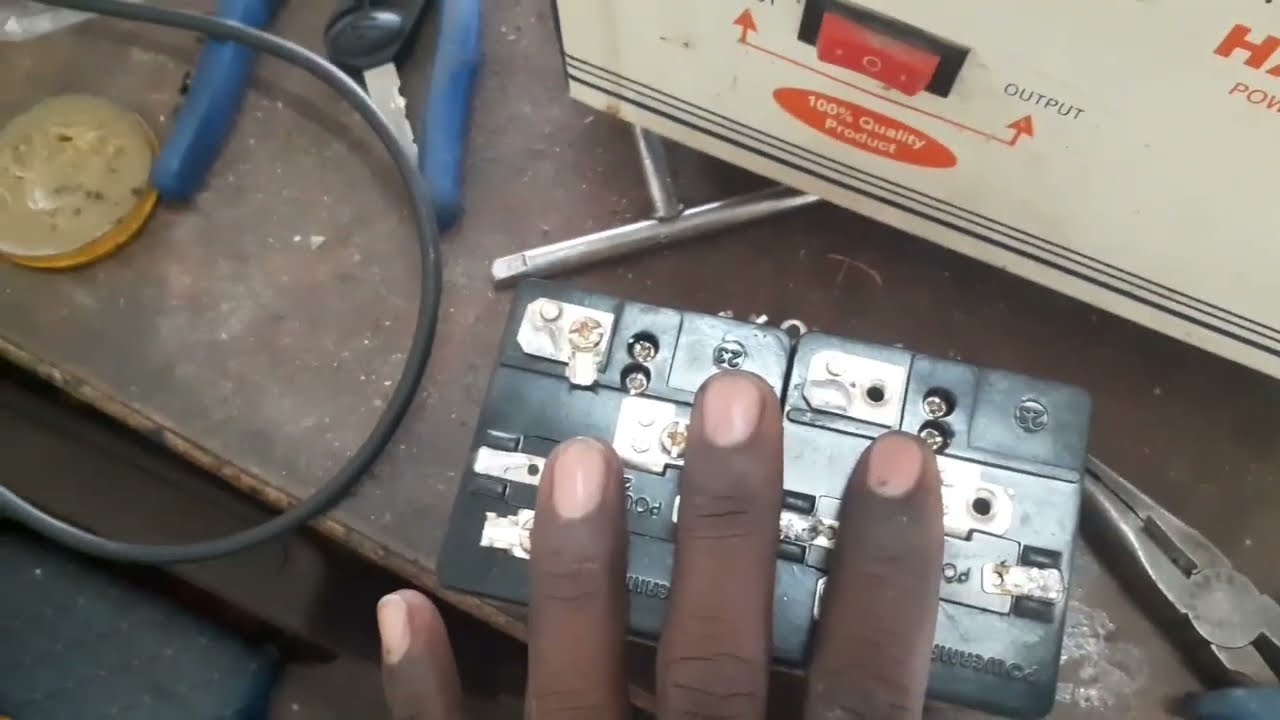The image, taken from a slightly elevated first-person perspective, captures a detailed view of a workbench. The focal point is a black person's left hand, with short-clipped fingernails painted soft pink, resting atop a thick, rectangular metal device with several small screws and partially visible text. The workbench is scattered with various tools: to the right of the hand lies a set of needle-nose pliers, while above and to the right, there is a white machine featuring an orange circle labeled "100% quality product" and a red toggle switch marked "output." Additional items include blue-handled pliers, a coiled black cable, a key, and other indistinct tools, suggesting a busy, tool-laden workspace. The surface of the workbench appears metallic, contributing to the industrious atmosphere.